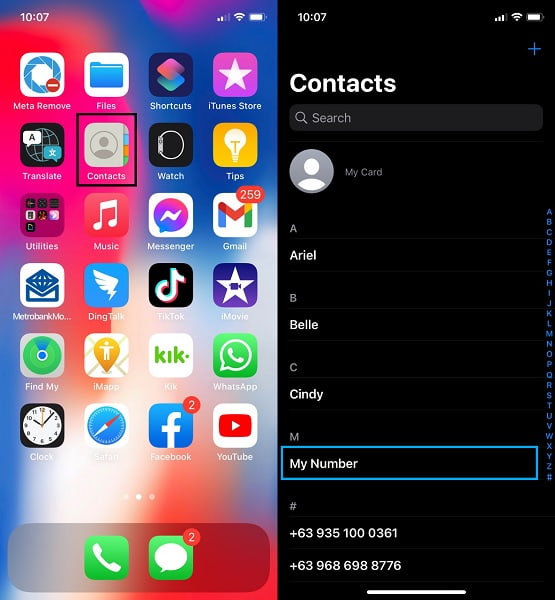The image comprises two screenshots. The first screenshot displays a mobile home screen with a predominantly blue background adorned with a few red and white blotches. The screen includes numerous app icons, such as Meta, Remote, Meta Remove, Files, Shortcuts, iTunes Store, Translate, Contacts (highlighted with a black square), Watch, Tips, Utilities, Music, Messenger, Gmail, MotorbankMO or MetrobankMO (the name cuts off), DingTalk, TikTok, iMovie, Find My, iMap, Keek, WhatsApp, Clock, Safari, Facebook (with a notification badge displaying the number 2), and YouTube. At the bottom of the screen are two icons: a green Phone icon and a green Message icon, with the Message icon also showing a notification number 2. Additionally, there's a numerical indicator "259" at the top of the screen, next to the network status "1007."

The second screenshot focuses on the Contacts app. It features a search bar at the top, followed by "My Card." Listed contacts include Ariel under "A," Belle under "B," Cindy under "C," and "My Number" under "M," which is highlighted with a blue rectangle.